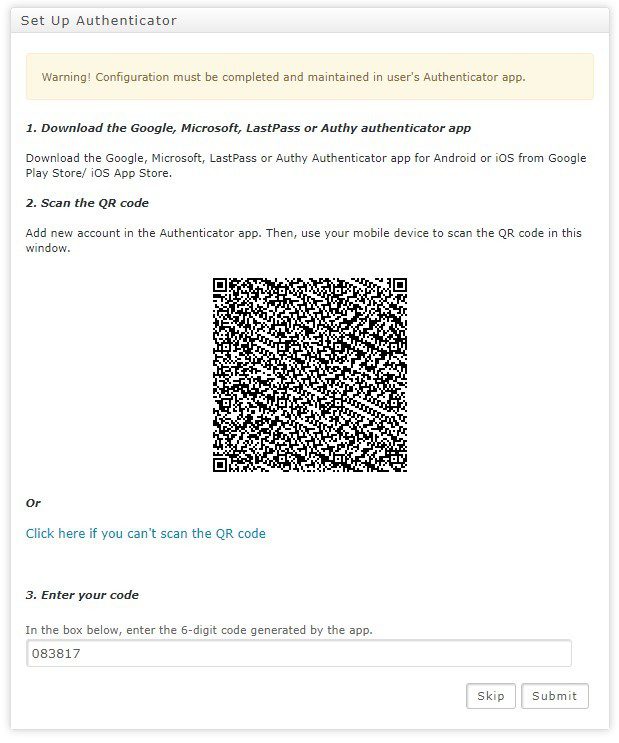Screenshot of the "Setup Authenticator" Interface:

The image displays the user interface of a Setup Authenticator tool. At the top, the title bar reads "Setup Authenticator," encapsulated by a thin gray border around the whole image. The background of the top section has a slightly colored hue, followed by a gray bar just below the title.

Central to the interface is a prominent yellow field bordered by light orange. This field contains the following warning message:
"Warning: Configuration must be completed and maintained by the Authenticator app."

Below this warning are detailed instructions presented in italicized text:
1. Download the Google, Microsoft, LastPass, or Authy Authenticator app for Android or iOS from the Google Play Store or iOS App Store.
2. Scan the QR code. It instructs users to add a new account in the Authenticator app and use their mobile devices to scan the QR code displayed in this window.

The QR code is located centrally and is quite large and busy. Underneath it, still in italics, there's a blue hyperlink reading: "Click here if you can't scan the QR code."

The final instruction:
3. Enter your code. Just above an input field, it says: "In the box below, enter the six-digit code generated by the app."

In the example provided within the input field, the code "083817" is currently entered.

At the bottom right-hand corner of the interface are two buttons—both white with a light gray outline. The left button is labeled "Skip," and the right button is labeled "Submit."